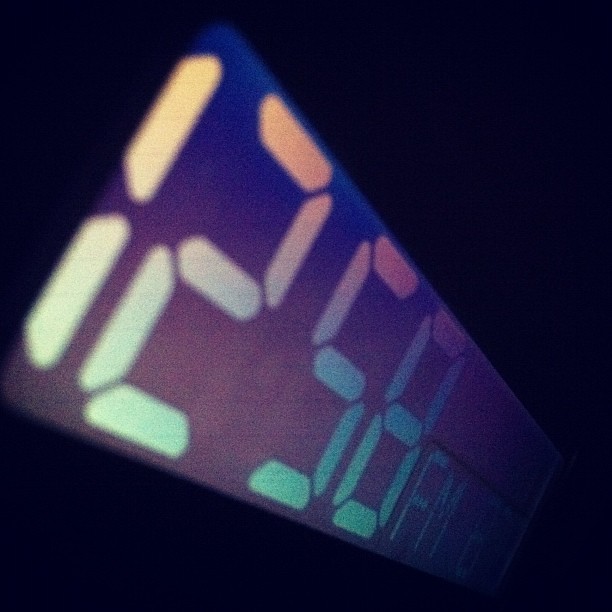This is a close-up photograph of a digital clock face, possibly an alarm clock, captured at a slight downward angle from the upper left to the lower right as if viewed from a bedside. The clock features a large LCD or backlit LCD screen with a dark blue-purple and grayish background. The display emits bright, fluorescent white neon light, making the numbers highly visible. The time appears to be 12:58, with the '1' in yellow, '2' transitioning from orange to green and yellow, '5' shifting from red to purple to blue and green, and '8' blending from purple to blue to green. There is some ambiguity about the exact indication, with another close number reading FM 87, which might be interpreted as a radio station setting. Surrounding the clock face, the image is completely pitch black, highlighting the vivid colors and emphasizing the bright, multicolored numerals.